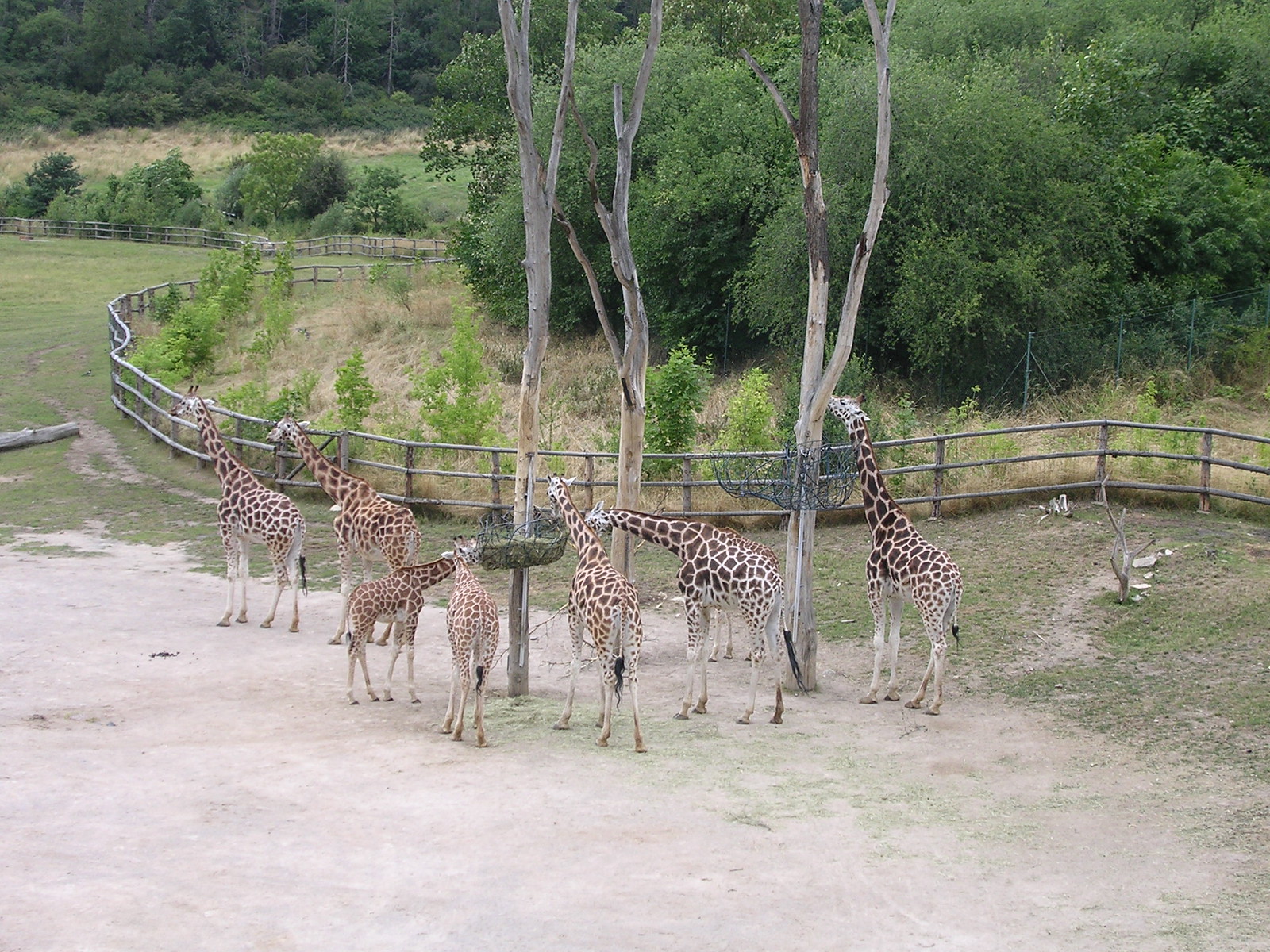This photograph captures seven giraffes in a zoo or wildlife reserve during feeding time, confined within a grassy enclosure bordered by a large fence. The giraffes are gathered around two tall, leafless trees that have wire baskets attached to their trunks. The main basket, filled with hay, is drawing the attention of the younger and smaller giraffes that are bending their long necks to feed. The larger giraffes, seemingly having already eaten, are moving away from the feeding spot. Notably, a secondary wire basket on another tree stands empty. In the background, a lush, green forest filled with tall trees provides a picturesque backdrop to the scene, contrasting with the more barren enclosure. The image vividly portrays the tranquil feeding routine of these majestic animals within their secure habitat.